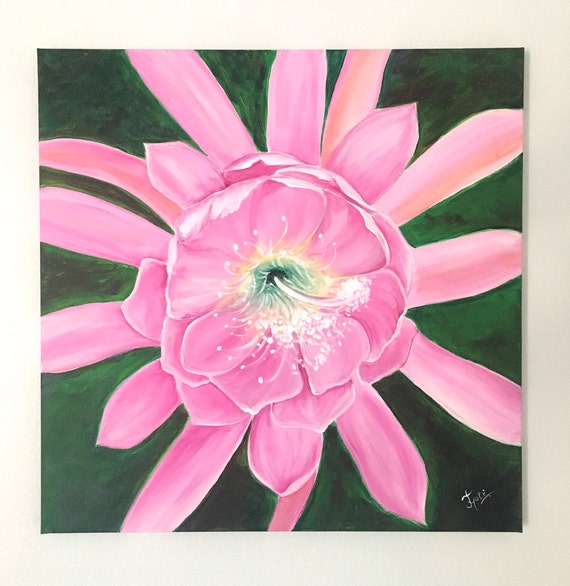The image is a meticulously detailed painting of a pink flower set against a green background. The painting, which is square-shaped, is so realistic that it takes a moment to realize it’s not a photograph. The artist has signed their name in white in the bottom right-hand corner. The flower is the focal point, prominently displayed in a zoomed-in perspective. It features numerous narrow, long petals that radiate outward from a central cluster. The innermost part of the flower has closer, larger petals, with green, yellow, and black hues and some white speckled pollen. The background, composed of various shades of green, provides a rich, contrasting backdrop that makes the pink petals pop. The painting captures the intricate details of the flower, including the pollen that appears to have settled on the petals, giving it a natural, textured appearance.